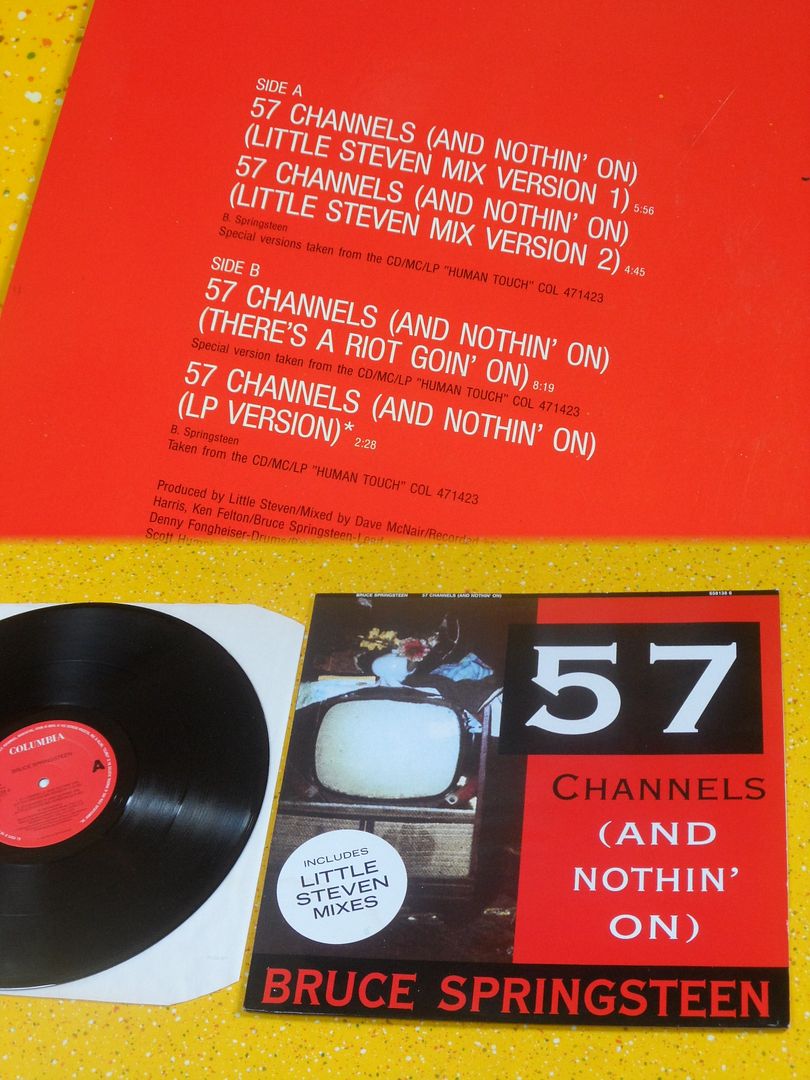The image depicts a colored print piece, likely part of an album cover, featuring three distinct sections. At the very top, there is a close-up of the back of Bruce Springsteen's record album titled "57 Channels (And Nothin' On)" from the late '80s or early '90s. The back cover, rendered in red with white print, lists the tracks and details such as Side A and Side B song titles, including "57 Channels (And Nothin' On)" remixed by Little Steven and the LP version of the song. Below this, much smaller and on the left, the LP record itself is displayed on its inner dust jacket, all set against a yellow countertop. The album cover features a small black and white TV screen illustration, representing "57 channels." A visible watermark from PhotoBucket reads, "Protect more of your memories for less."